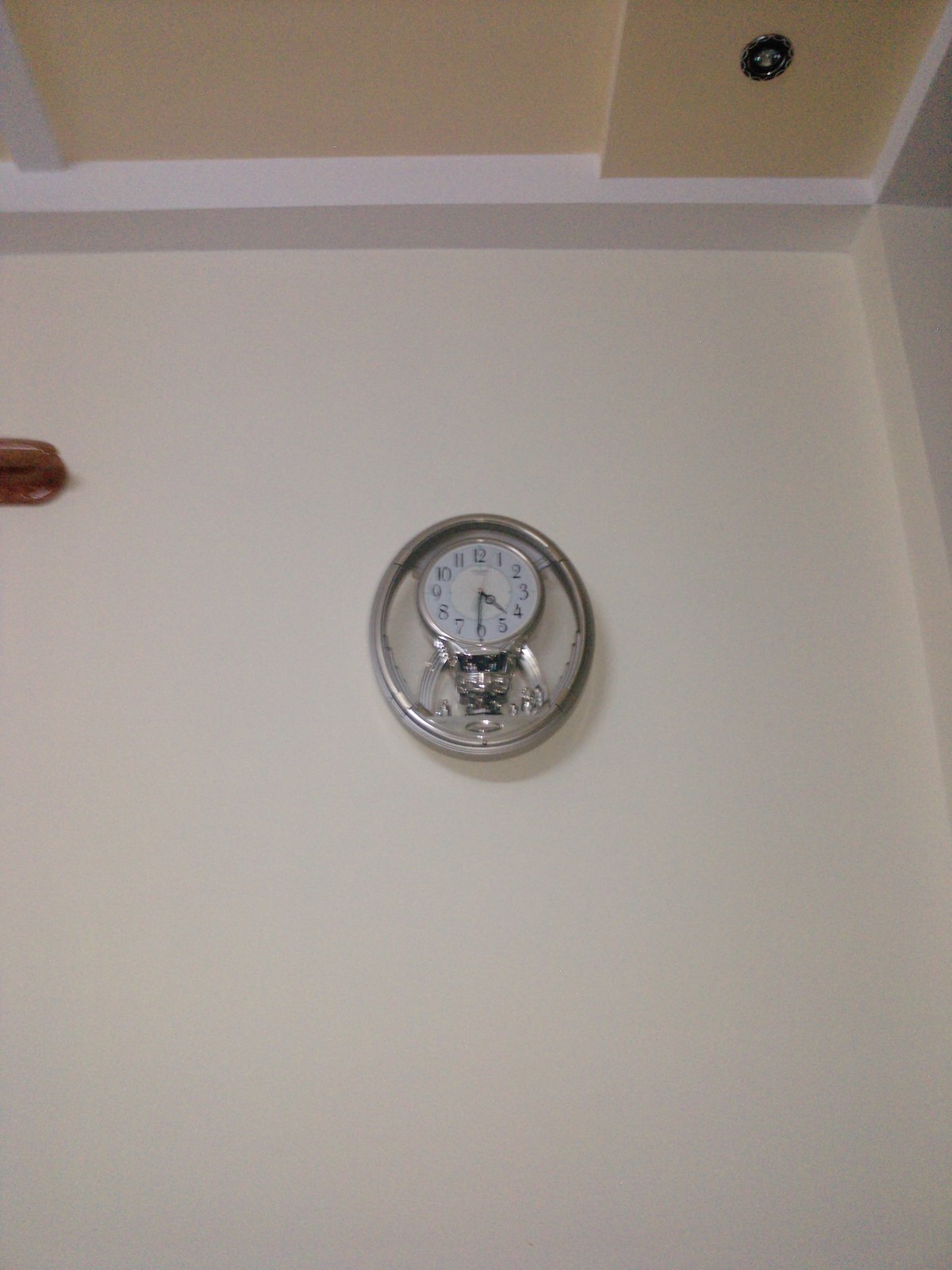This color photograph captures a meticulously designed clock mounted on a white wall. The clock features a white face adorned with bold black numerals from 1 to 12 and is equipped with black hour and minute hands. Although the second hand’s color is indiscernible, its presence is suggested. The clock is encased in a sophisticated silver metal frame, with a glass cover providing protection over its face.

Distinctively, the clock sits within an oval-shaped stainless steel ring that contributes to its aesthetic appeal. This metal ring is not a perfect circle but more of an oval, accentuated with a silver point at the bottom and two silver legs extending from the face outward to the ring, providing structural support. The entire setup appears to be slightly elevated on four grommets, giving it a raised appearance above its circular base. 

The clock is set at approximately 4:30, casting a subtle shadow on the pristine white wall behind it. The background is predominantly white, with tannish yellow sides that could be interpreted as the ceiling edges stepping down. Additional details include a brown object at the upper left and various architectural elements like an eggshell white post on the right wall, and a white line traversing the ceiling on the left side, enhancing the intricate setting of the scene.